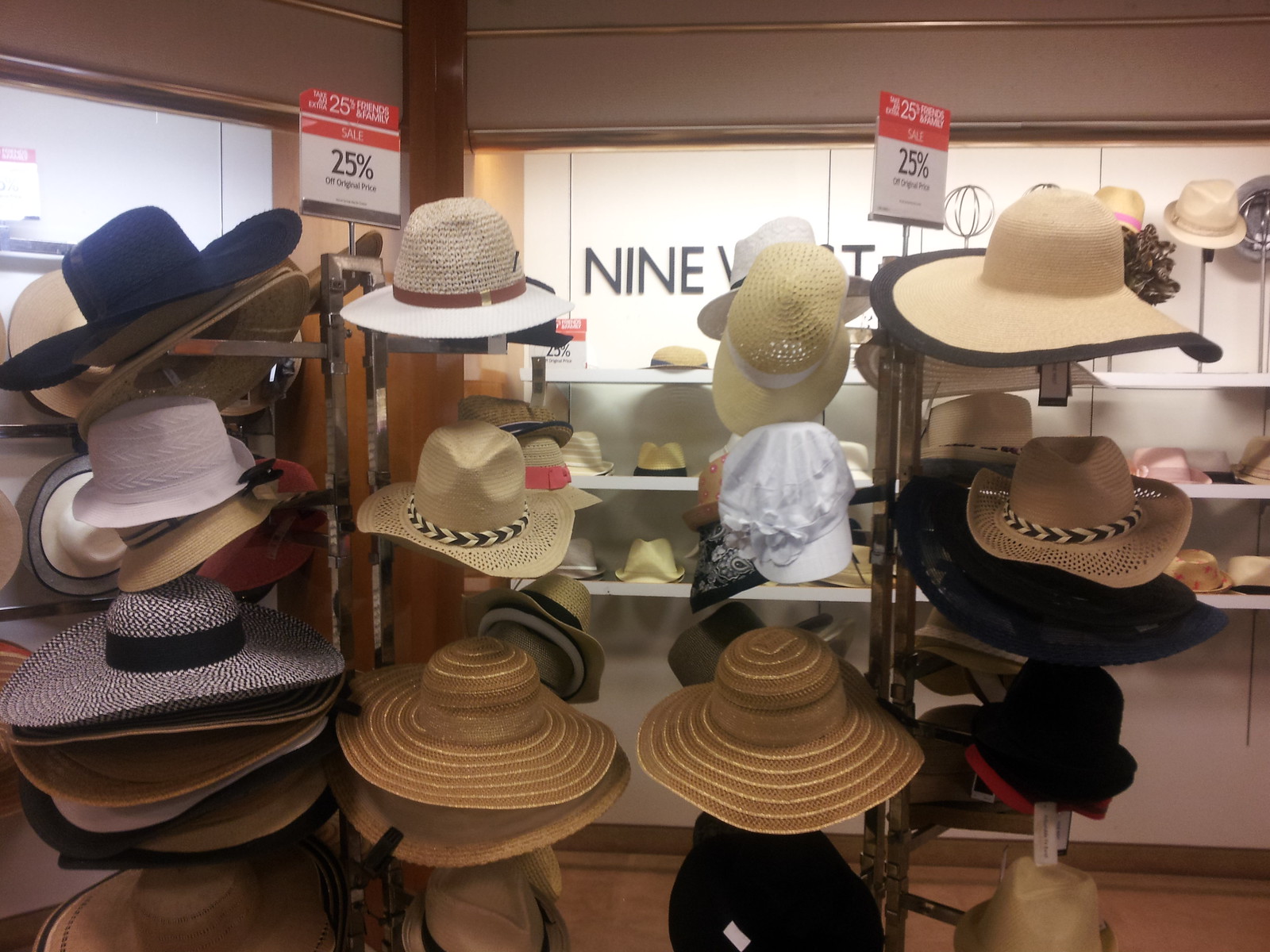This image captures an interior scene of a department store focused on hat displays. Dominating the foreground are two vertical, silver metal racks adorned with numerous hats. These racks are marked by red and white signs proclaiming "SALE" and "25% OFF," indicating a discounted offer. The hats come in a variety of styles, including wide-brimmed sun hats typically made of wicker material, taller cowboy-styled hats, and a few fedoras. Predominantly, the hats are in neutral tones such as beige, brown, and black, with some variation in their shading.

The background features white shelves arranged in three horizontal levels against a wall, each shelf showcasing individual hats. The central wall sports a sign emblazoned with "9 WEST" in dark brown capital letters on a white backdrop. The adjacent left wall, tinged in light pink with gold borders, also holds additional hat displays, though the specifics are less discernible. The floor appears to be brown, complementing the overall aesthetic. 

Additionally, the scene includes a distinctive black brimmed hat, a white brimmed hat, and a black-and-white brimmed hat among the more traditionally colored headgear. The meticulous arrangement and variety of hats, along with the promotional signage, vividly convey a bustling retail environment devoted to headwear.